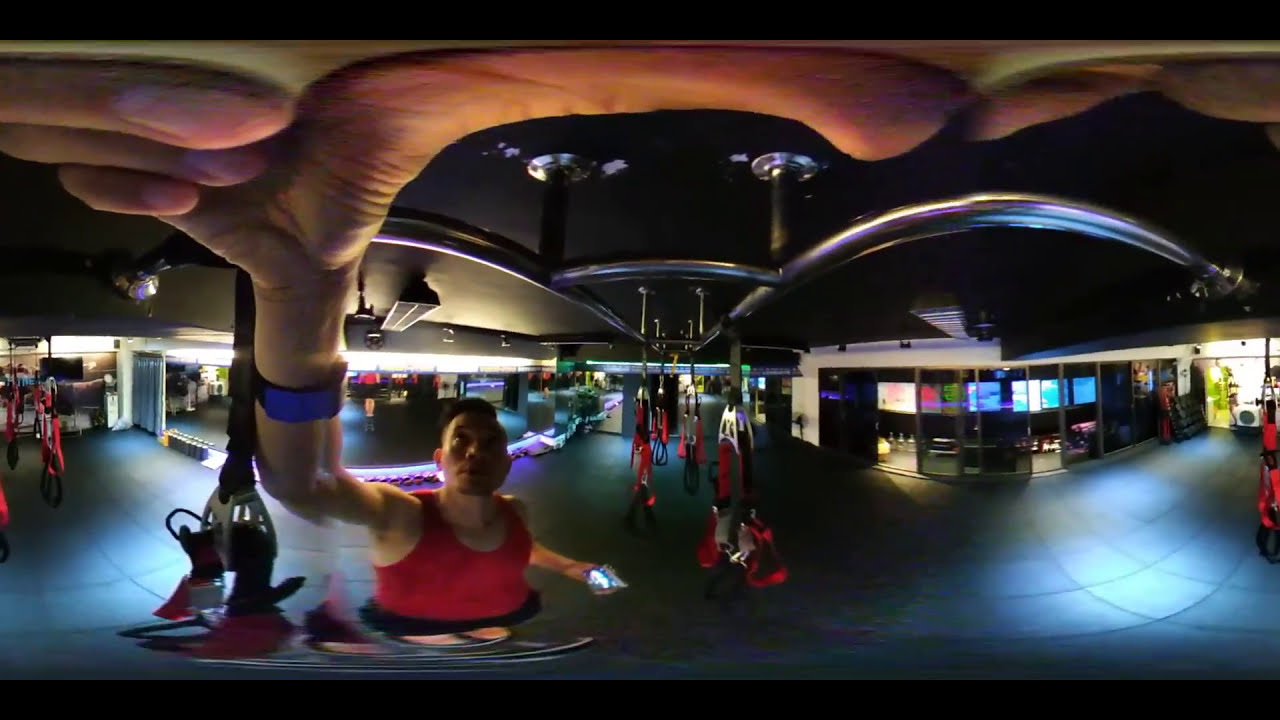The photograph captures the interior of a gym or sports studio, featuring a dark tile floor and an almost black ceiling with chrome bars. Dominating the center-left of the image is a man wearing a red tank top and black shorts, holding a camera with his right hand stretched upwards, causing his hand to appear comically large and superimposed over the top of the photograph. A blue device is seen on his wrist. In his left hand, he appears to be holding a cell phone. Surrounding him, the gym is equipped with various workout stations, mirrors, and metal railing systems with harnesses—a setup likely for calisthenics or similar exercises. The ceiling supports multiple handles or bands for workouts. To the left, a wall-length mirror reflects the gym’s interior, while to the right, a room with sliding glass doors and multiple television screens displaying red, white, and blue colors can be seen, contributing reflections that light up the dark floor.